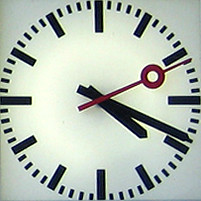The image depicts a minimalist analog clock featuring a white background with black lines and dashes in place of numbers. The clock has three hands: a short hour hand, a longer minute hand, both black, and a red second hand distinguished by a small red circle near its base. The hour markers are represented by thicker black lines, with slightly thinner lines denoting the five-minute intervals, and even thinner lines for the individual minutes. The time displayed on the clock is approximately 4:18. The clock's overall design is simple and utilitarian, reminiscent of those commonly found in middle schools.